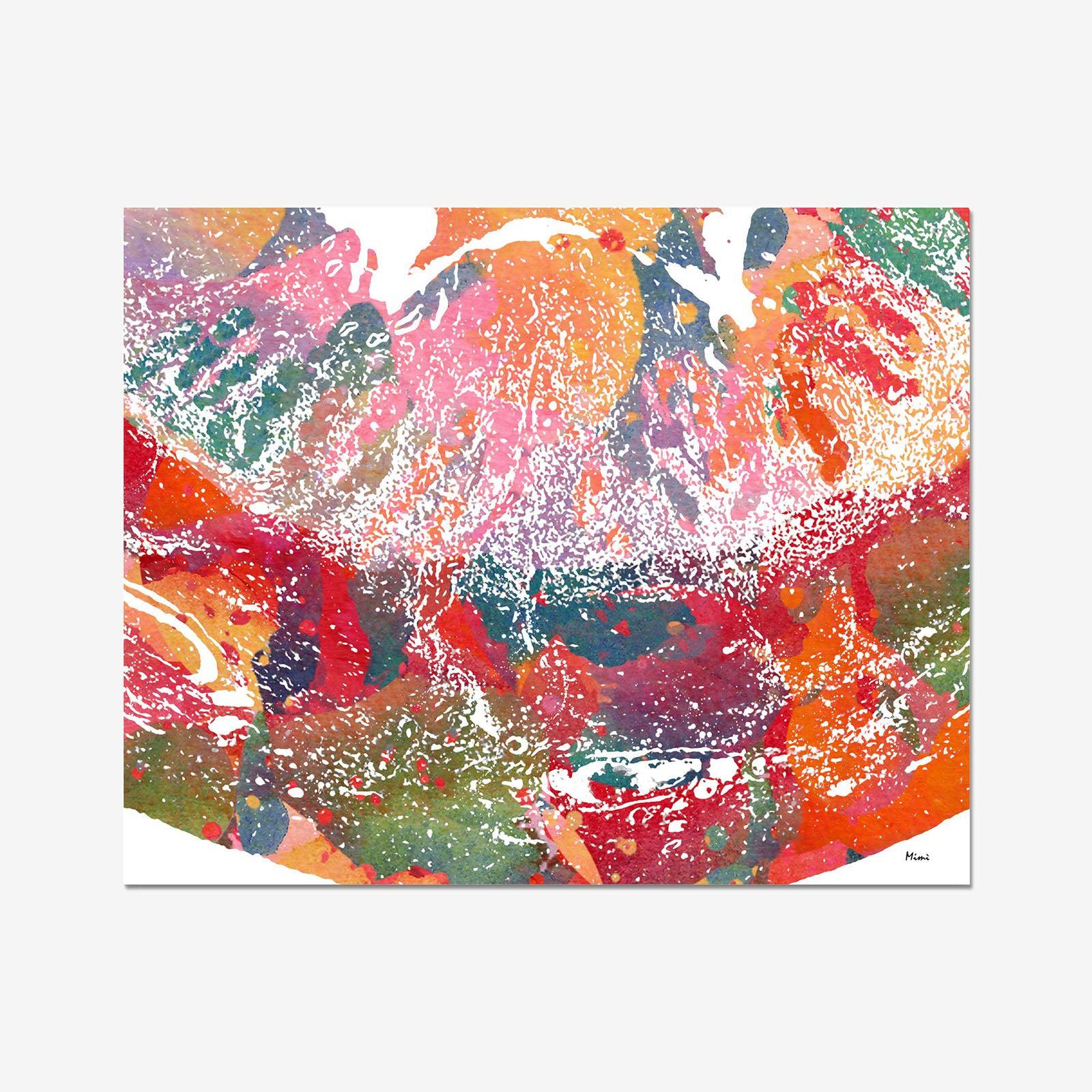The image is a vibrant piece of artwork that appears to be a digital mock-up of a painting displayed on a white wall, casting a subtle drop shadow. The painting incorporates an array of dynamic colors, including orange, red, green, blue, and pink, applied in splotches and blobs, resembling watercolor or sponge paint techniques. The composition features a swirling, almost pointillist design pattern, covered with areas of white paint that mimic the look of seafoam or rippling water. The edges of the artwork are marked by more saturated colors, transitioning to pastel, speckled whites towards the center. Despite the abstract nature and lack of a particular design, the entire piece is framed against a clean white background with a subtle autograph in the corner, adding a touch of personal flair.